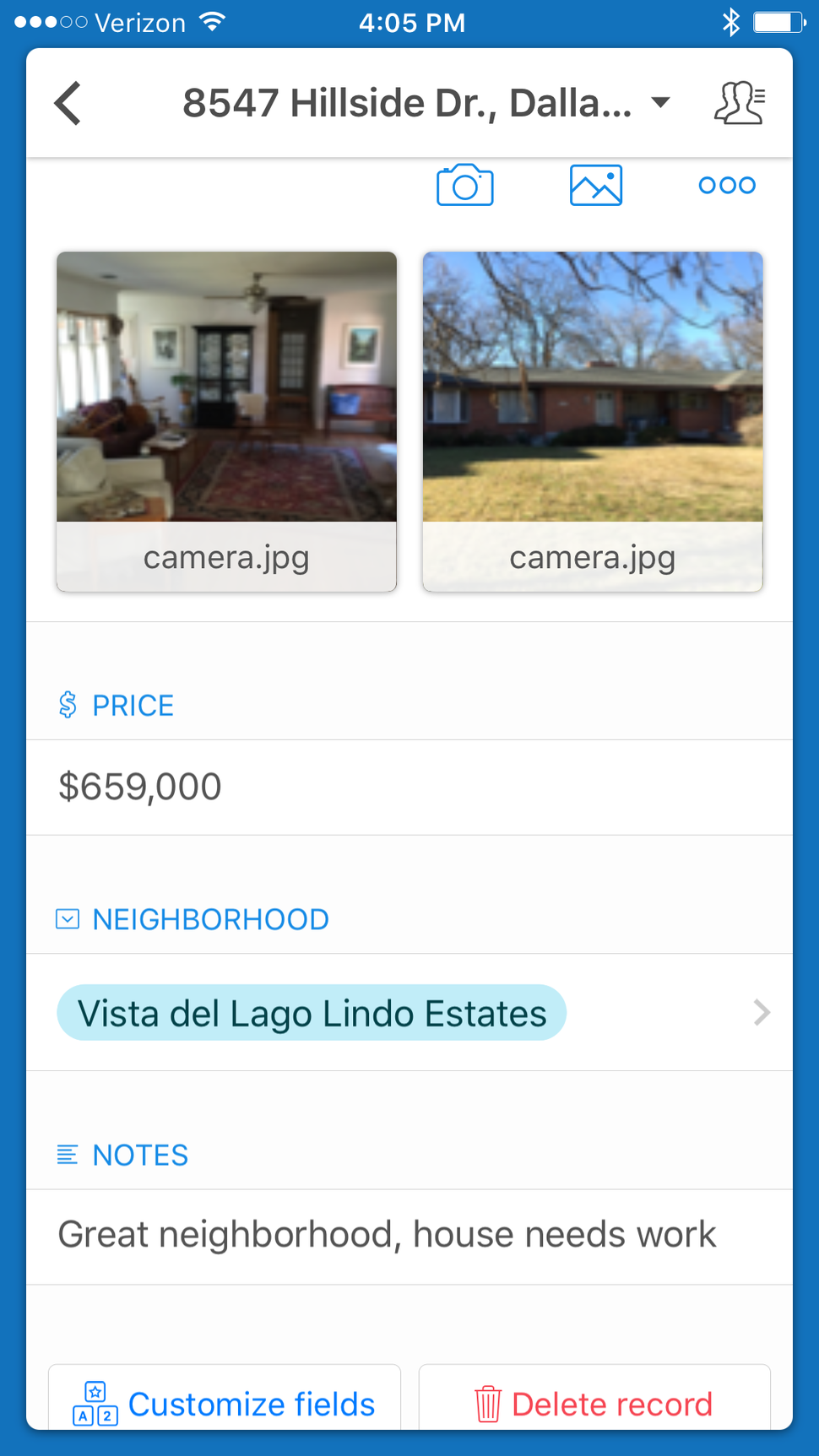The image showcases a search result page for a real estate property displayed on a user's cell phone. The screen indicates it's 4:05 PM, the device is on the Verizon network, and the battery is nearly full. The interface is a white vertical rectangle set against a dark blue background.

At the top of the screen, "8547 Hillside Drive" is prominently written in black, indicating the property is located in Dallas, Texas (though the word 'Dallas' is partially cut off). Below this, there are icons for calling, photos, and additional options (three dots) highlighted in blue.

The layout features two side-by-side images: one of a living room interior and the other of the property's exterior taken from the yard. The asking price for the home is prominently displayed as $659,000.

Further down, the page lists "Neighborhood" in light blue, followed by a light blue button stating "Vista Del Lago Lindo Estates." Under the "Notes" section, also in light blue, it reads "Great Neighborhood House Needs Work."